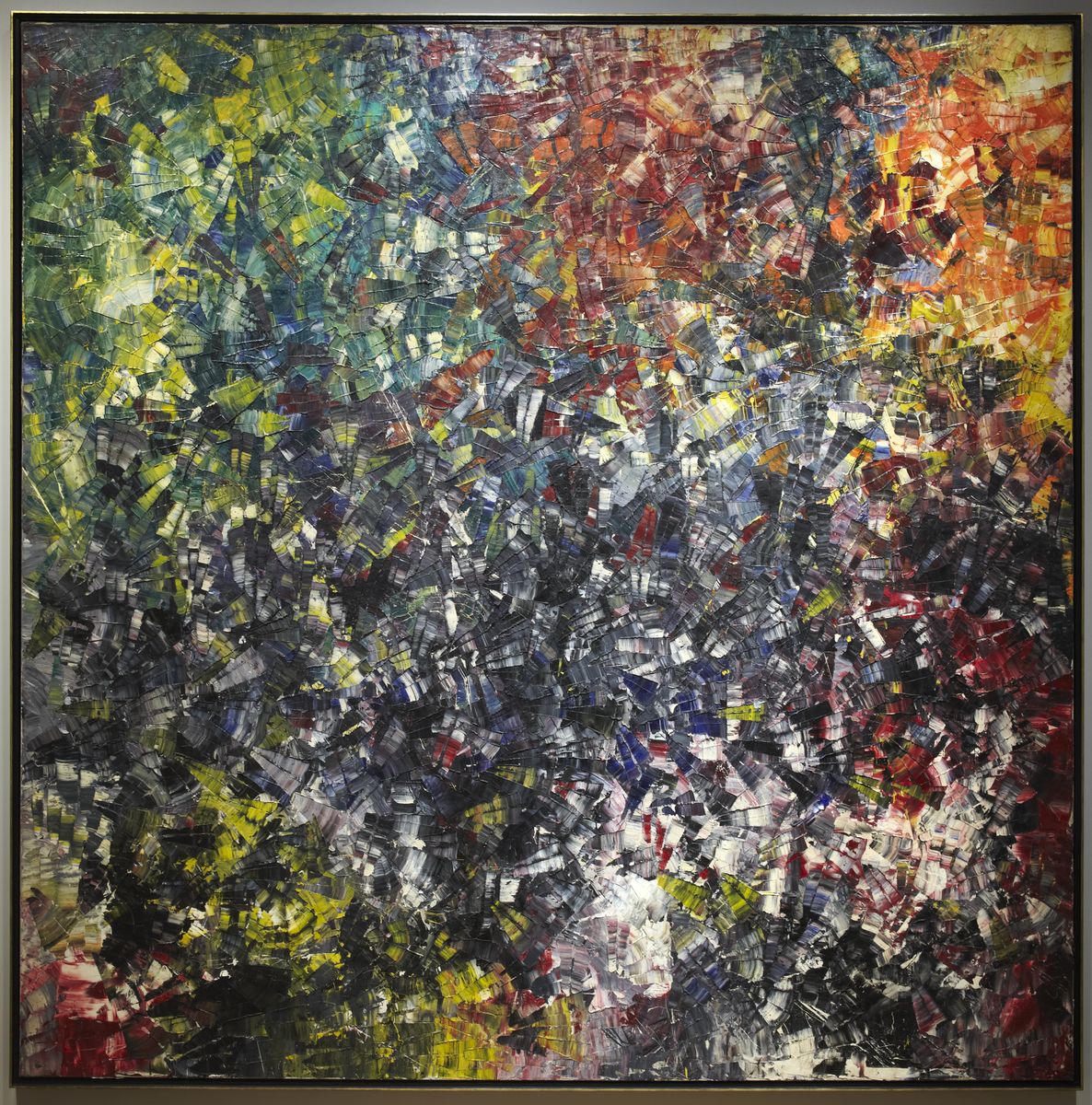This artwork is a highly abstract painting characterized by a choppy and thick application of paint, almost as if the artist attacked the canvas with their brush. The piece is composed of hundreds of small, trapezoidal shapes, predominantly with corners and edges, creating a collage or mosaic-like facade. The colors are meticulously sectioned and organized, with the center featuring dark hues interspersed with touches of white. Moving outwards, the top middle transitions to red, the middle right to orange, and the bottom right to a mix of black and red. The bottom of the canvas is predominantly white, while the bottom left integrates red, black, and yellow. The top right corner is dominated by yellow shades, and the top left is filled with dark green, green-yellow, and light blue tones. Despite the varied colors, the overall tone of the painting is dark and subdued, with each hue containing deeper, more somber tones. The composition leaves an impression reminiscent of an autumn day, perhaps symbolizing a bowl of fruit or flowers, capturing an array of emotions and abstract forms.